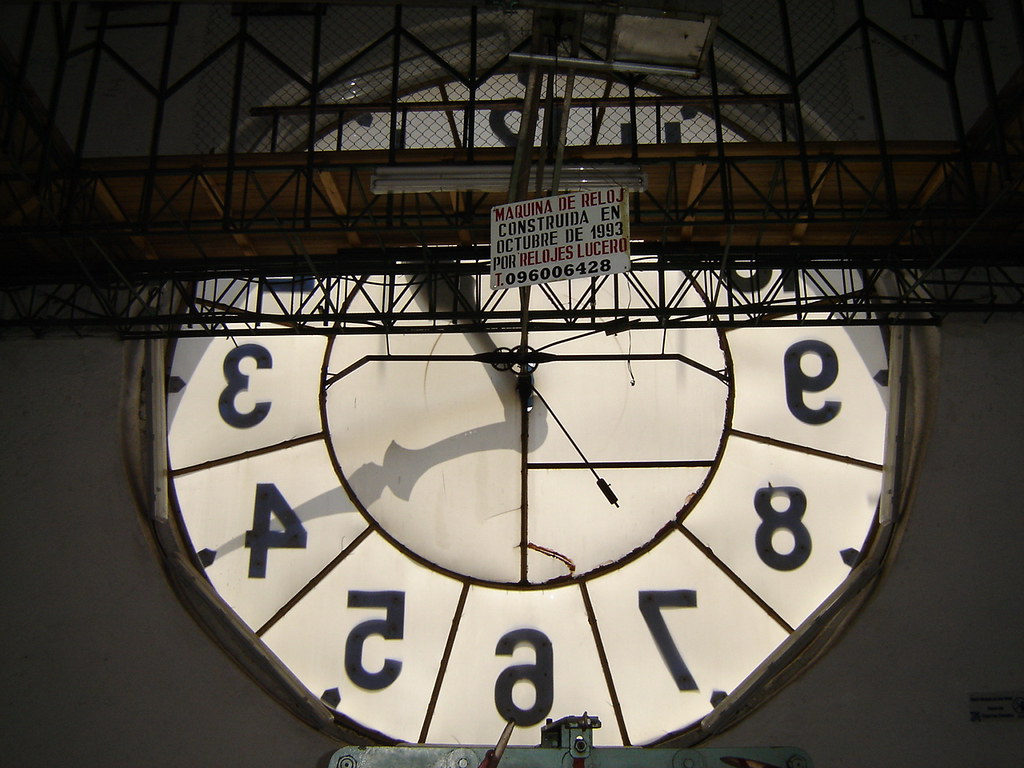The photograph depicts the intricate interior of a clock tower with a towering, oversized clock face dominating the background. The clock, viewed from behind, features inverted numbers ranging from 3 to 9, casting shadows from the hands onto the clock face. The scene is framed by modern, sans-serif structural elements and a black fence in the foreground. This fence holds a white sign with red and black lettering, reading "máquina de reloj, máquina de reloj construida octubre de 1993 por relojes lucero" along with a phone number, 096-00-642-8, providing a historical context in Spanish. The backdrop presents a gradient gray sky, lighter at the bottom and darker at the top, adding to the dramatic atmosphere of the image. Near the clock, there appears to be equipment used by constructors, possibly for maintenance or access, hinting at ongoing interaction with this impressive timekeeping mechanism.